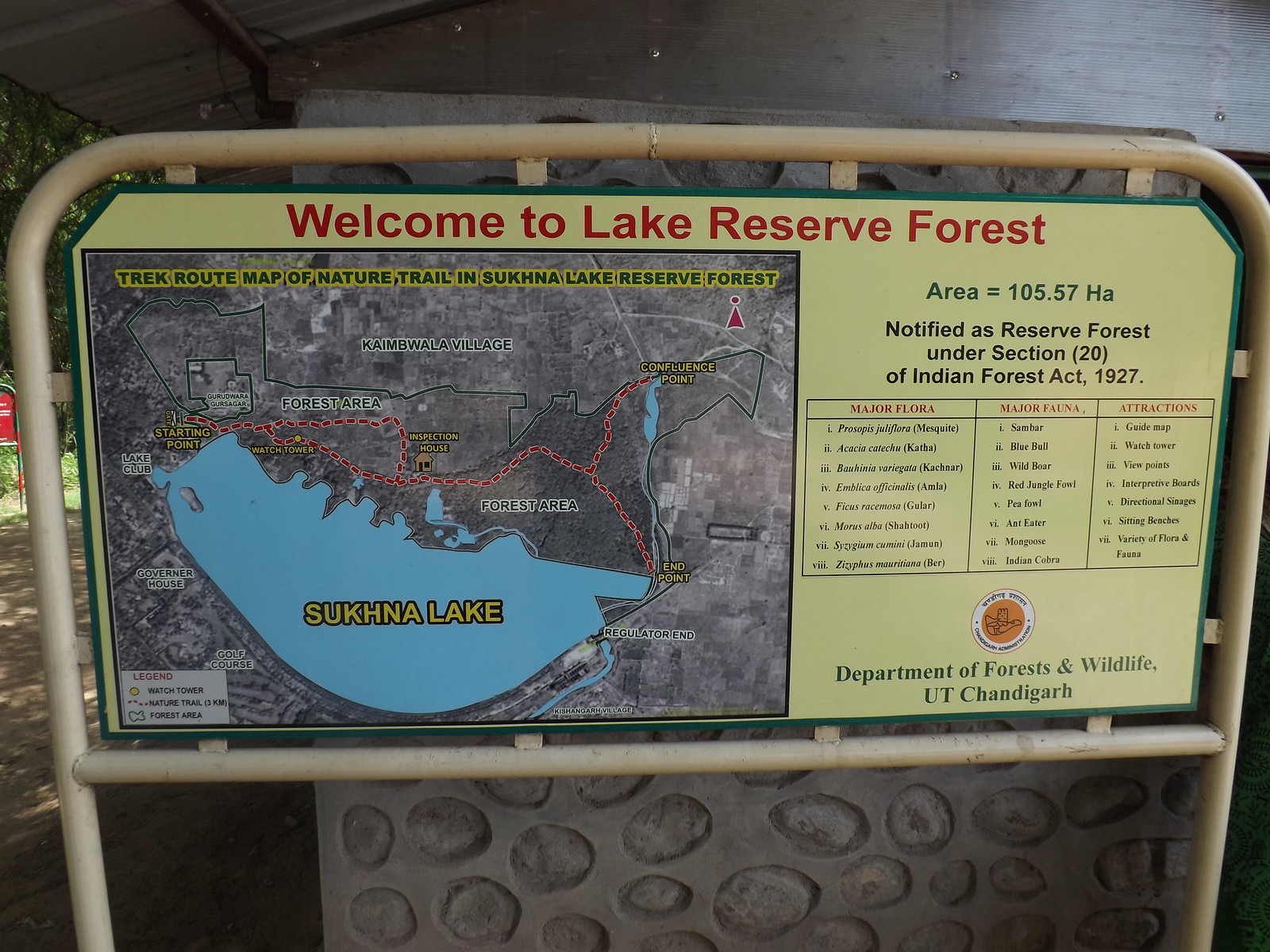This horizontally aligned rectangular picture features a detailed sign mounted on light brown metal poles, resembling a guardrail, that curve to form a rectangular bracket. The sign, suspended within this structure, possesses a light green background with a darker green border, and is prominently displayed in an outdoor setting. 

At the top of the sign, large red letters proclaim, "Welcome to Lake Reserve Forest." Below, a map illustrates the "Trek Route Map of the Nature Trail in Sukhna Lake Reserve Forest," with a blue depiction of Sukhna Lake at its center. Surrounding the lake are labeled land areas including Kainbwa Village, forest area, endpoint, confluence point, and start point. The map is detailed with red dotted lines indicating the route of the trail.

To the right of the map, the sign provides additional information stating, "Area = 105.57 HA, Notified as Reserve Forest under Section 20 of Indian Forest Act 1927." Beneath this, a chart with three columns highlights "Major Flora," "Major Fauna," and "Attractions," presented with red headings and black text. 

At the very bottom, green letters read, "Department of Forests and Wildlife UT Chandigarh." The background includes trees with green leaves and partial views of covered areas with sheet metal roofing, indicative of a serene natural setting.